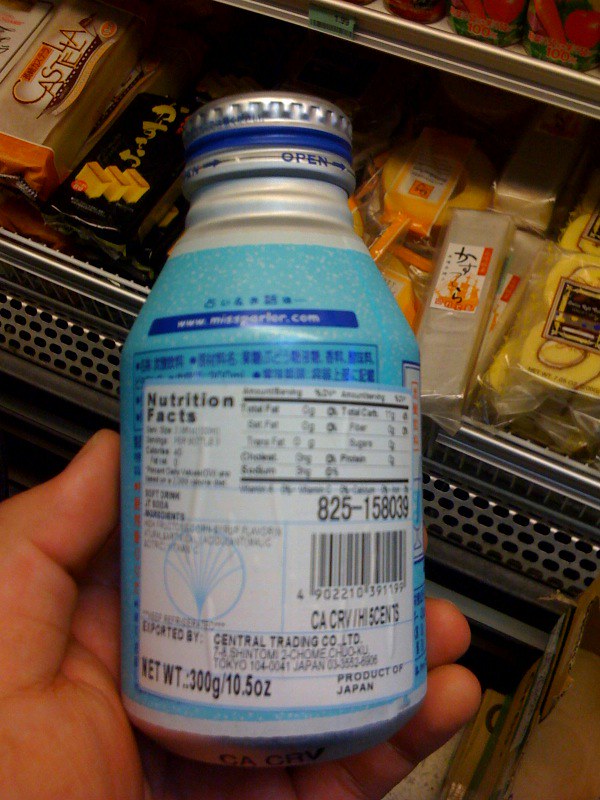A high-resolution photograph captures a hand holding a small product bottle against a background filled with various packaged items.

The image centers on the hand, showcasing only the fingers and the thumb, with the wrist just out of the frame. The hand firmly grasps a light blue bottle, approximately palm-sized, featuring dark blue nutritional information printed directly on it.

A white, rectangular sticker with nutritional facts in English is affixed over the original text, concealing the foreign language underneath, which appears to be either Chinese, Japanese, or Korean. The bottle also bears a circular blue stamp with intricate lines, possibly a logo or certification mark. The bottle is capped with a distinctive silver lid marked by a blue stripe.

In the background, a cluttered basket brims with various food products, hinting at a market or store setting. The packaging, predominantly adorned with Japanese characters, indicates their origin, and among the items, a package resembling cinnamon rolls can be discerned. The overall scene is vibrant and bustling, emphasizing the product amidst a plethora of Asian food items.